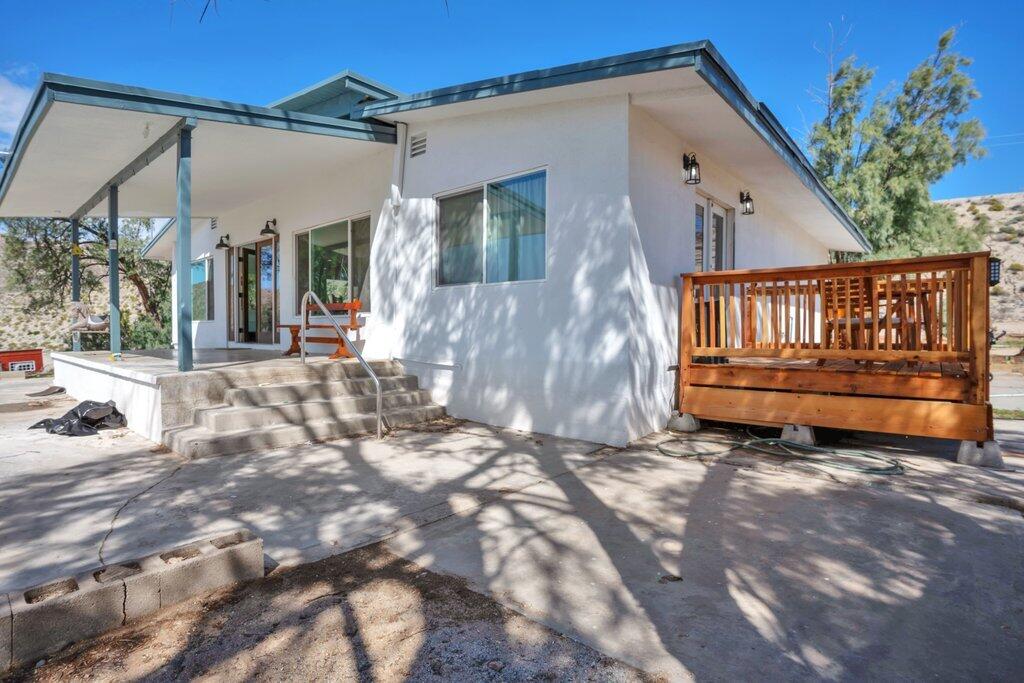This image depicts a single-story white stucco house in a desert-like environment, possibly resembling locations in California, Arizona, or Nevada. The house is set against a backdrop featuring a mostly clear blue sky, a small cloud on the left, and a distant hill with patches of dirt stretching to the skyline. Flanking the house are trees that cast shadows on the structure and the ground.

Prominent in the foreground is a reddish-brown wooden deck on the right side, elevated on concrete blocks and adorned with a patio door flanked by two outdoor wall sconces. The deck features seating with visible chairs and a green hose coiled on the ground beside it. The front of the house is characterized by a small raised concrete porch accessible via four steps with a chrome-colored central handrail. The porch, which faces left, is supported by three blue vertical pillars and has an overhang extending approximately four feet. An orange bench sits on this porch, adding a touch of color.

The central door on the porch is flanked by two double windows on each side and a triple window to its right, providing symmetry to the facade. The roof appears to be blue, complementing the blue trim and supports on the porch. The yard surrounding the house is predominantly concrete, forming an L-shape and framing the house with no presence of grass, aligning with the desert aesthetic. The concrete extends to the right side and beneath the deck, further emphasizing the arid environment portrayed in the photograph.